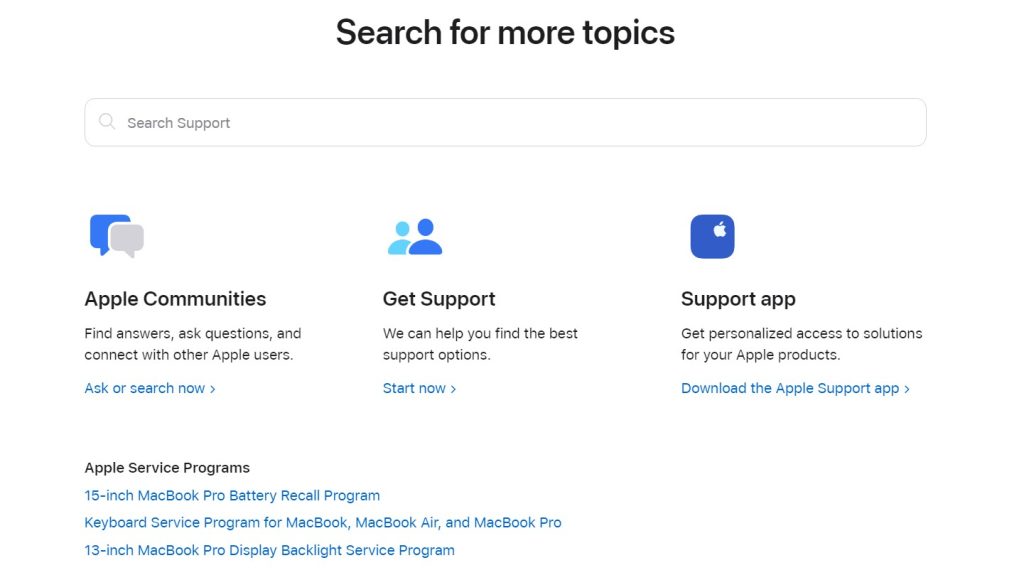The image depicts a search screen from an Apple support webpage. It is horizontally oriented, featuring a predominantly white background that seamlessly blends into the content area.

At the top, the header reads "Search for more topics," followed by a central search bar with the placeholder text "Search Support" in gray. This allows users to type in queries for assistance.

Below the search bar are three columns, each featuring a blue icon aligned to the left. The columns are titled "Apple Communities," "Get Support," and "Support App." 

- "Apple Communities" includes a description: "Find answers, ask questions, and connect with other Apple users." A blue hyperlink beneath this column invites users to "Ask or search now."
- "Get Support" likely provides options for users to obtain direct assistance for their issues, though specific text for this is not given.
- "Support App" probably guides users to download or use the support application for their devices.

Further down, the section labeled "Apple Service Programs" highlights three important service initiatives, each presented as a blue hyperlink. These are:
1. "15-inch MacBook Pro Battery Recall Program"
2. "Keyboard Service Program for MacBook, MacBook Air, and MacBook Pro"
3. "13-inch MacBook Pro Display Backlight Service Program"

The overall layout is clean and user-friendly, aiding seamless navigation for Apple users seeking support or information about service programs.